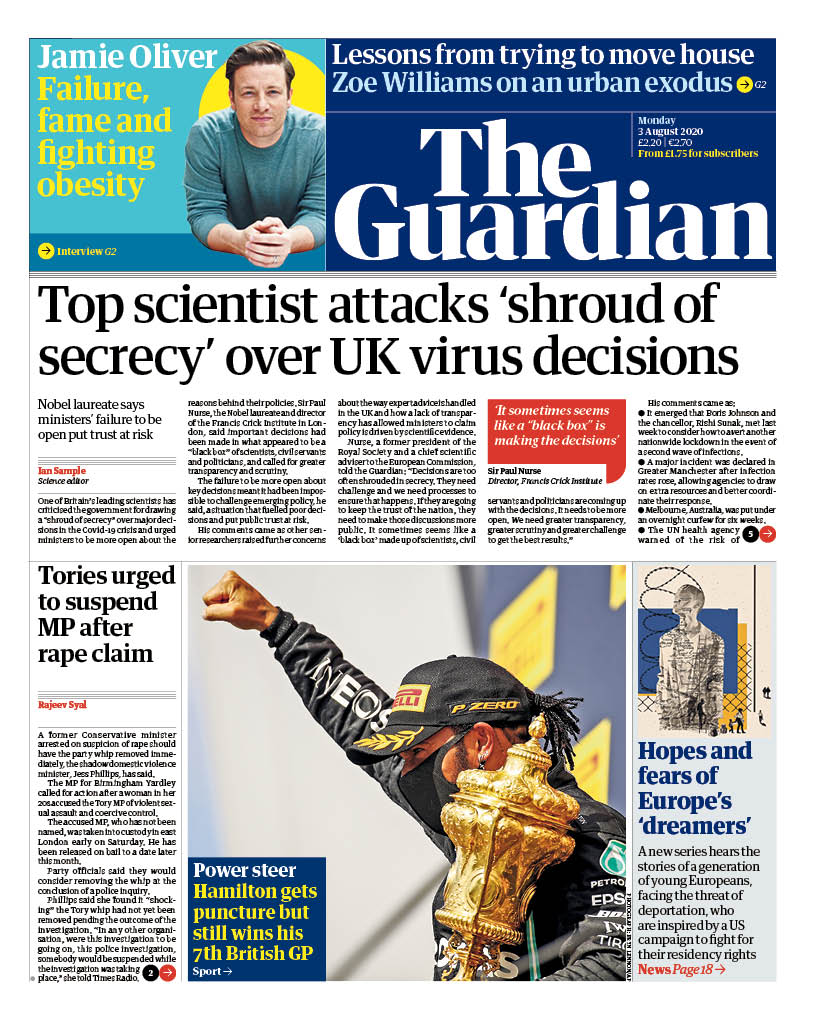The image captures the front page of The Guardian newspaper, which has a traditional newspaper layout. At the top of the page, there are two prominent sections side by side. The smaller section on the left features an article titled "Jamie Oliver: Failure, Fame, and Fighting Obesity," accompanied by a photograph of Jamie Oliver. In the image, Oliver, a man with brown hair wearing a long-sleeve shirt, faces the camera with his hands extended in front of him.

The larger section on the right has a headline at the top stating "Lessons from Trying to Move House: Zoe Williams on an Urban Exodus." Below this headline, in larger white font, is "The Guardian," indicating the publication. The date, Monday, August 3rd, 2020, is visible beneath the newspaper's title.

Spanning both sections at the top, there is a main headline reading, "Top Scientists Attack Shroud of Secrecy Over UK Virus Decisions," underscoring a leading story about criticism from scientists regarding the UK's handling of virus-related information.